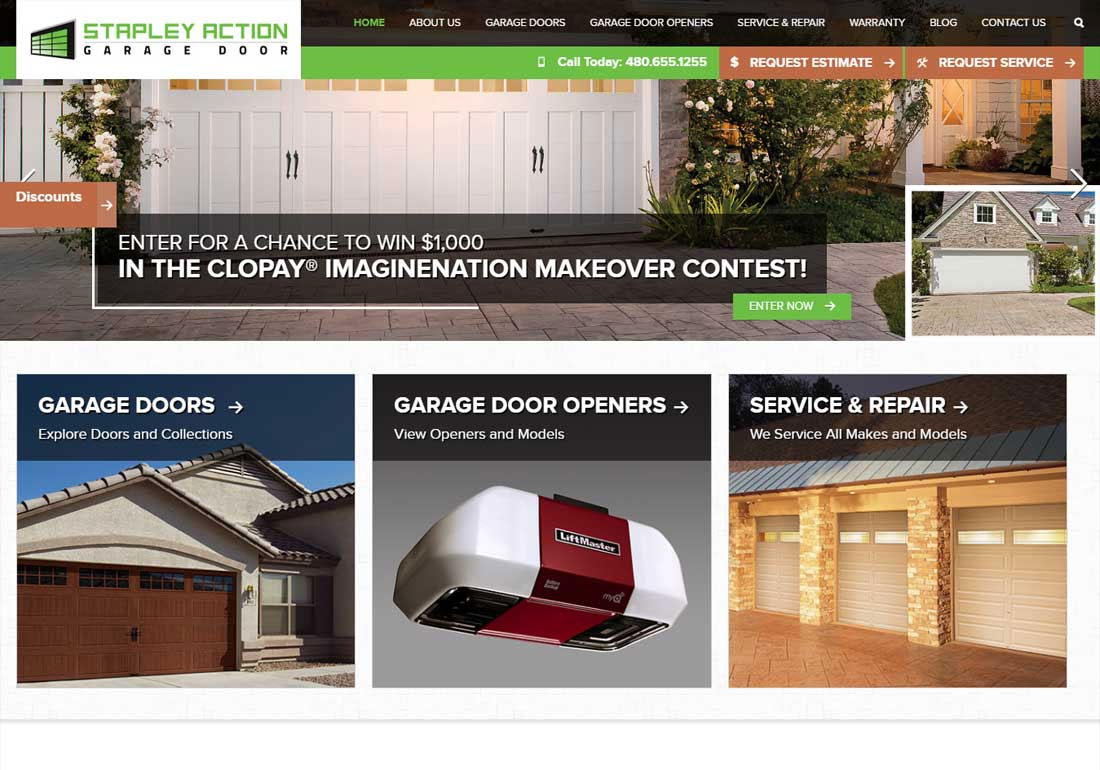This is a color image taken from the website of Stapley Action Garage Door, a company specializing in garage door installation. In the top left corner, the website showcases their green garage door logo with the words "Stapley Action" also written in green. The navigation bar provides several options including Home, About Us, Garage Doors, Garage Door Openers, Service and Repair, Warranty, Blog, and Contact. Additionally, there is a search function for the entire site.

The website encourages visitors to call their service number, 480-655-1255, or utilize buttons to request an estimate or services. A prominent red button labeled "Discounts" is also visible on the page.

Central to the page is an announcement for the Clopay Imagination Makeover Contest, accompanied by a green "Enter Now" button. The background image features two aesthetically pleasing garage doors, and a smaller adjacent image displays a recently installed large garage door on an upscale home.

At the bottom, three colorful, clickable tabs offer additional options: 
1. "Garage Doors" - presenting a brown garage door with options to explore doors and collections.
2. "Garage Door Openers" - showcasing a white and red unit, with options to view openers and models.
3. "Service and Repair" - highlighting that the company services all makes and models of garage doors.

The layout and images collectively emphasize the quality and range of services provided by Stapley Action Garage Door.